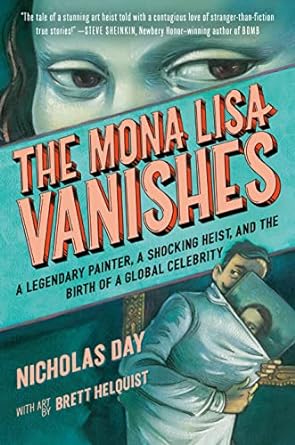This detailed book cover features a striking illustration with a dominant blue and white color scheme. At the top, in small, white text, it reads: "The tale of a stunning art heist told with the contagious love of stranger than fiction true stories. —Steve Sheinkin, Newbery-winning author of Bomb." Below this, the cover displays a large, close-up image of the Mona Lisa from her eyes upward, showing her eyes and part of her hair and forehead.

A diagonal light blue banner runs across the cover from the left center to the upper right, with bold pink letters stating: "The Mona Lisa Vanishes." Below this, in black text, it reads: "A legendary painter, a shocking heist, and the birth of a global celebrity."

At the bottom of the cover, there's a detailed drawing of a man with dark hair and a mustache, wearing a white coat. He appears to be concealing the Mona Lisa under his jacket, with part of the painting visible. The bottom left corner of the cover has the text: "Nicholas Day with art by Brett Helquist."